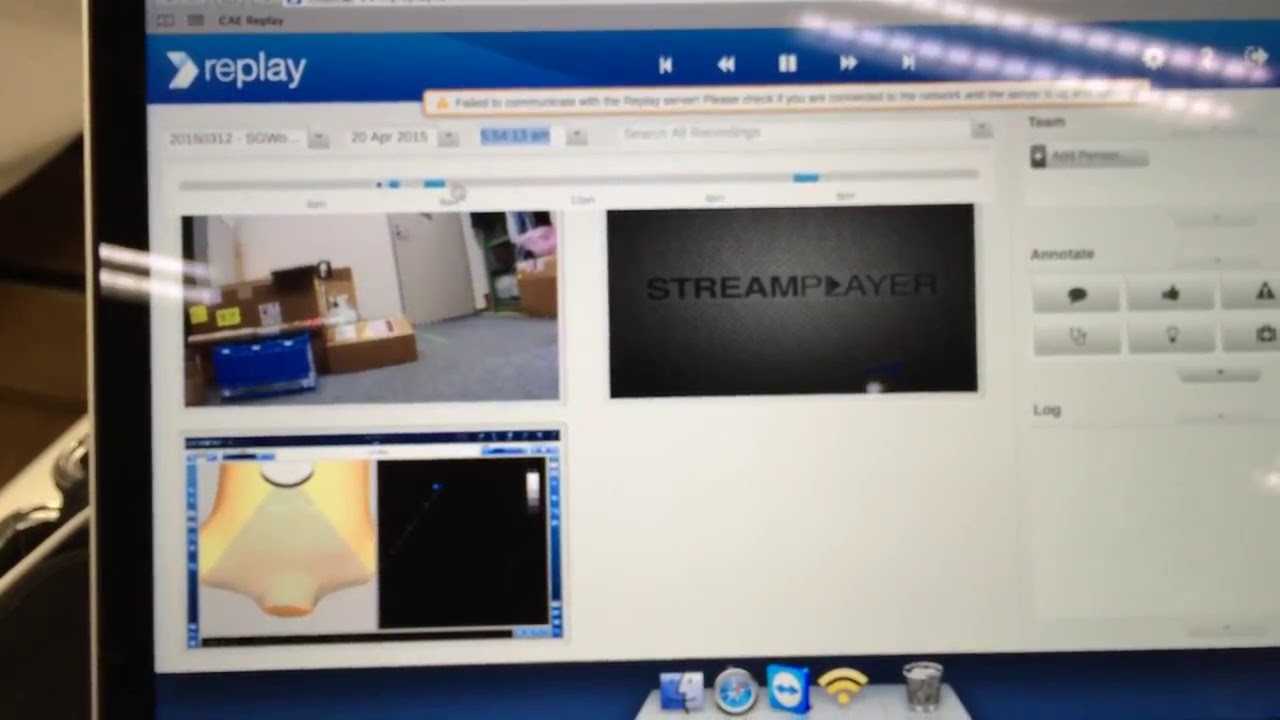This image captures a close-up photograph of a Mac computer screen, prominently centered and occupying the majority of the frame, suggesting the setting is a home office. On the screen, a web browser window is open displaying a website interface titled "Replay," identifiable by a blue bar with white letters and a right-pointing arrow logo on the left. The interface features three distinct sections: one shows the floor of an office with visible boxes and a door, another section labeled "Stream Player" appears grayed out, and the third shows what looks like a split view—one part depicting a yellow bowl and the other a black screen. Various on-screen controls and menus are visible on the right side. At the bottom of the screen, the familiar Mac dock displays icons for Task Manager, Safari, and the Trash Can. The photo includes several colors such as tan, black, brown, silver, blue, yellow, and gray, with a few indistinguishable objects to the left side of the monitor.